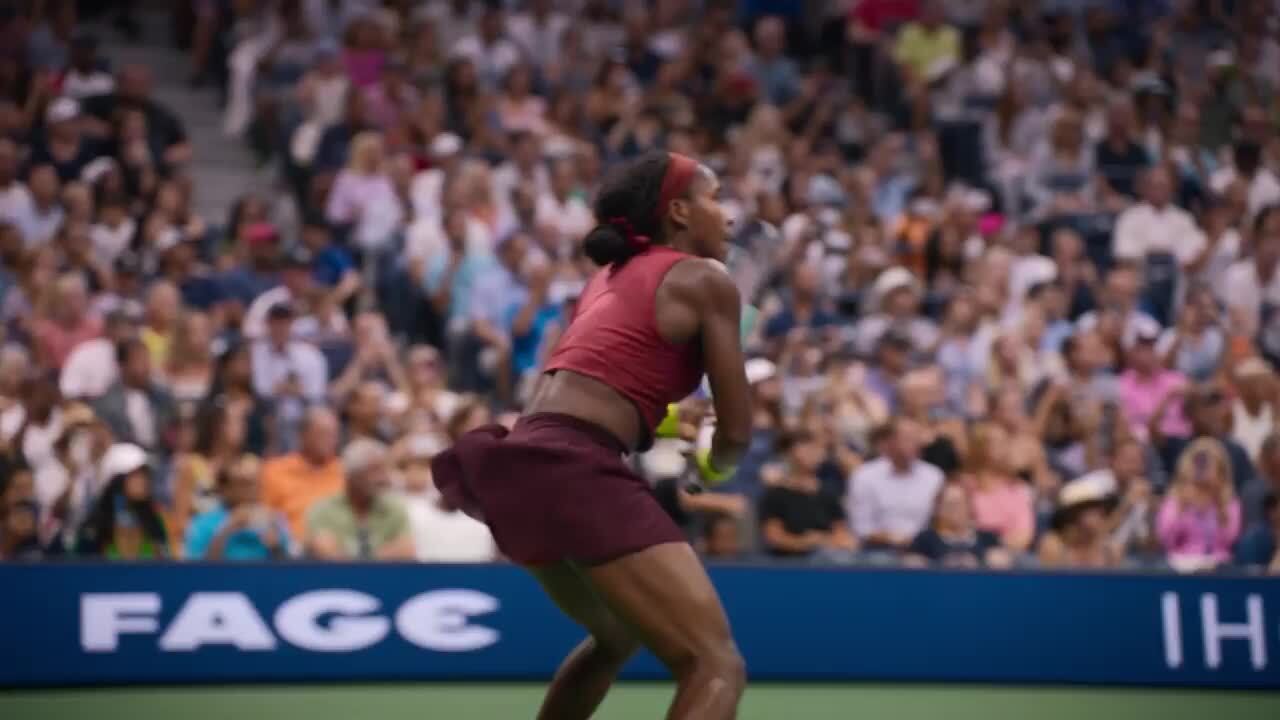The image depicts a dynamic scene from a live-action tennis match featuring a female tennis player, possibly Venus Williams. Captured from behind, she is poised in mid-motion with a racquet in hand, her bent knees suggesting imminent action. She sports a maroon tennis skirt paired with a reddish, sleeveless crop top, complemented by a matching headband positioned above her forehead. Her athletic ensemble is rounded out with brown and yellow athletic shoes and white socks. She has brown hair and a dark skin tone, identifying her as African-American. The court surface is blue with green surrounding areas, typical of a hard court. In the background, a packed stadium reveals rows of spectators in various colored outfits, with banners promoting brands like FAGE and IHG adorning the blue barricade at the court's edge.